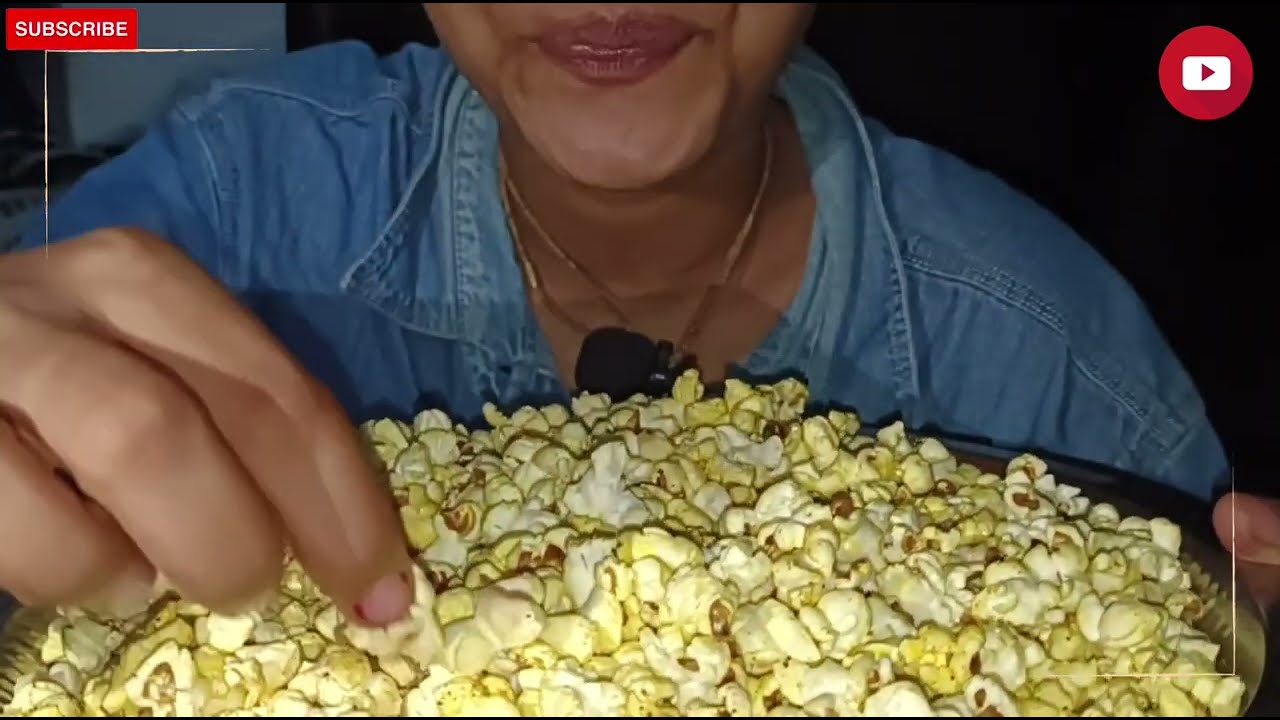This detailed image captures a still from a YouTube video prominently displayed in the top left corner with a red "Subscribe" button. On the top right corner, a red circle with a white play button signifies the YouTube icon. The focus of the image is a close-up of a person, likely a woman, wearing a collared denim shirt and two gold necklaces. Her face is partially visible, revealing pink lipstick and lips pursed as she reaches into a large, black bowl brimming with yellow and white buttered popcorn. The person's left hand holds the bowl, while the right hand dips in to grab some popcorn. The scene exudes a sense of enjoyment, as the person appears to be filming themselves eating from the ample bowl of popcorn. The background features mostly muted tones, highlighting the colors of the shirt, skin, and popcorn.